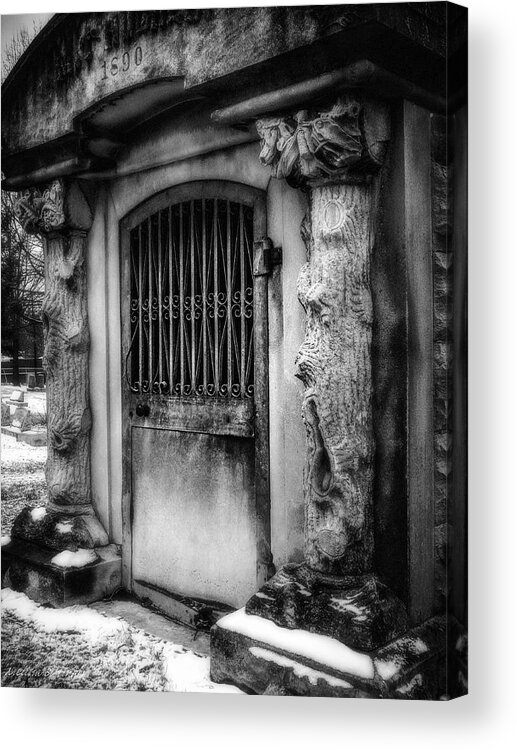The image depicts a tall, rectangular, black-and-white photograph of what appears to be the front entrance of an 1890s mausoleum. The structure features a metal door adorned with a zigzag grate on its upper half and visible door handles. The building is crafted from concrete stone and framed by two carved pillars that resemble trees with intricate ribbon designs near their tops and hollow bases. These columns, almost Greek-like in their detail, appear to support the small awning overhead, which prominently displays the year "1890." There is snow covering the ground and the lower portion of the structure, as well as some snow on the trees and grass visible to the left. The entire scene has a weathered, somewhat dirty appearance, adding to its historical ambiance. Unreadable white writing is noticeable in the bottom left corner, and a small canvas side segment is visible on the right, giving a hint of depth to the image.